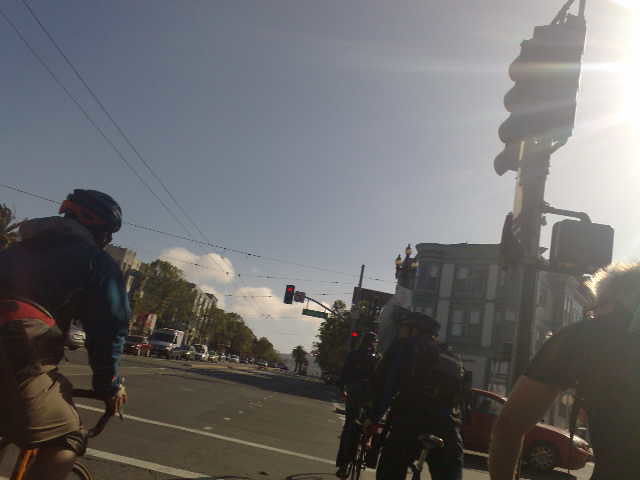The photograph captures a city intersection bustling with activity, viewed from the perspective of a cyclist. At the forefront, there are several cyclists: one closely positioned on the right edge of the image, two directly ahead, and another on the left. They are waiting at a set of traffic lights. The nearest traffic light is prominently featured on the right side, with a red sedan visible driving across the intersection in the background. Further in the distance, additional traffic lights span across the street. The background is punctuated by urban buildings lining both sides of the street. On the left side, a row of cars is queued, facing towards the viewer, while lush green trees frame the scene, adding a touch of nature to the urban landscape.